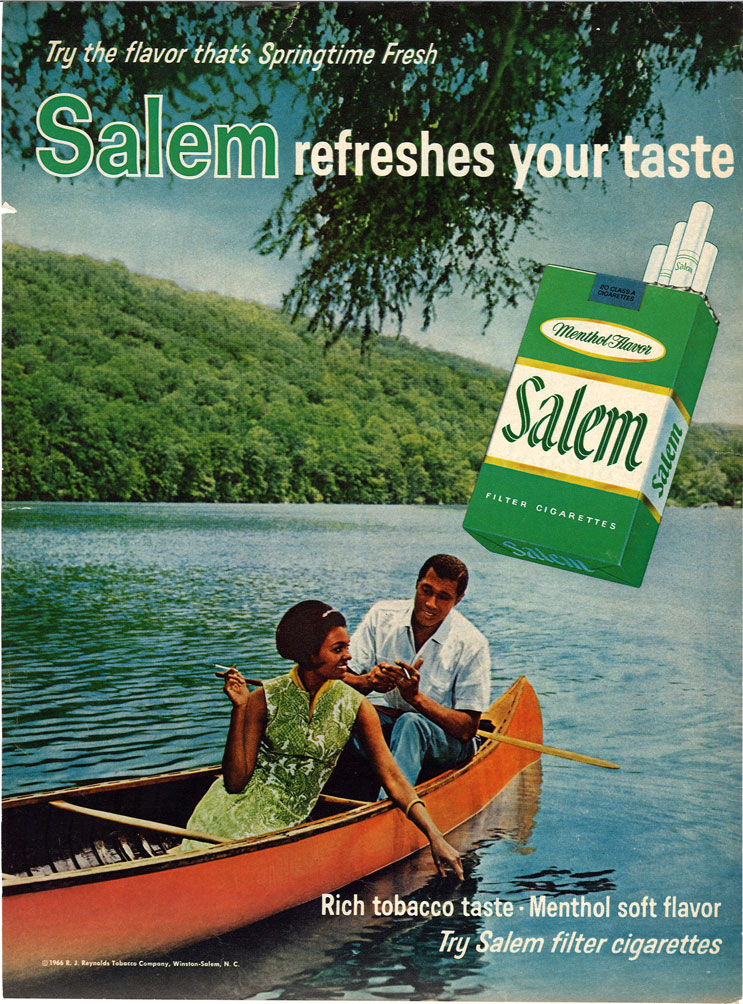This detailed image captures a vintage magazine advertisement for Salem Filter Cigarettes, prominently featuring a couple leisurely seated in a red rowboat on a tranquil lake surrounded by a forested landscape with hills rising in the background. The woman, an African American, is positioned towards the center of the boat, wearing a green dress with white accents, short black hair, and a white headband. She is holding a cigarette in her right hand and touching the water with her left. The man, a white individual, is seated at the edge of the boat behind her, dressed in a short-sleeved white dress shirt and blue dressy pants. Both appear to be engaged in conversation, each holding a cigarette.

To the right side of the couple, a large floating pack of Salem Filter Cigarettes dominates the scene with its distinctive green packaging, gold and white accents, and images of individual cigarettes emerging from the pack. Above the pack, the text reads, "Try the flavor that's springtime fresh. Salem refreshes your taste," with 'Salem' written in large green letters with a white outline. At the bottom of the advertisement, beneath the boat, are the words, "Rich Tobacco Taste, Menthol Soft Flavor. Try Salem Filter Cigarettes." The background is completed by a sky overhead and a dense array of trees lining the shore.